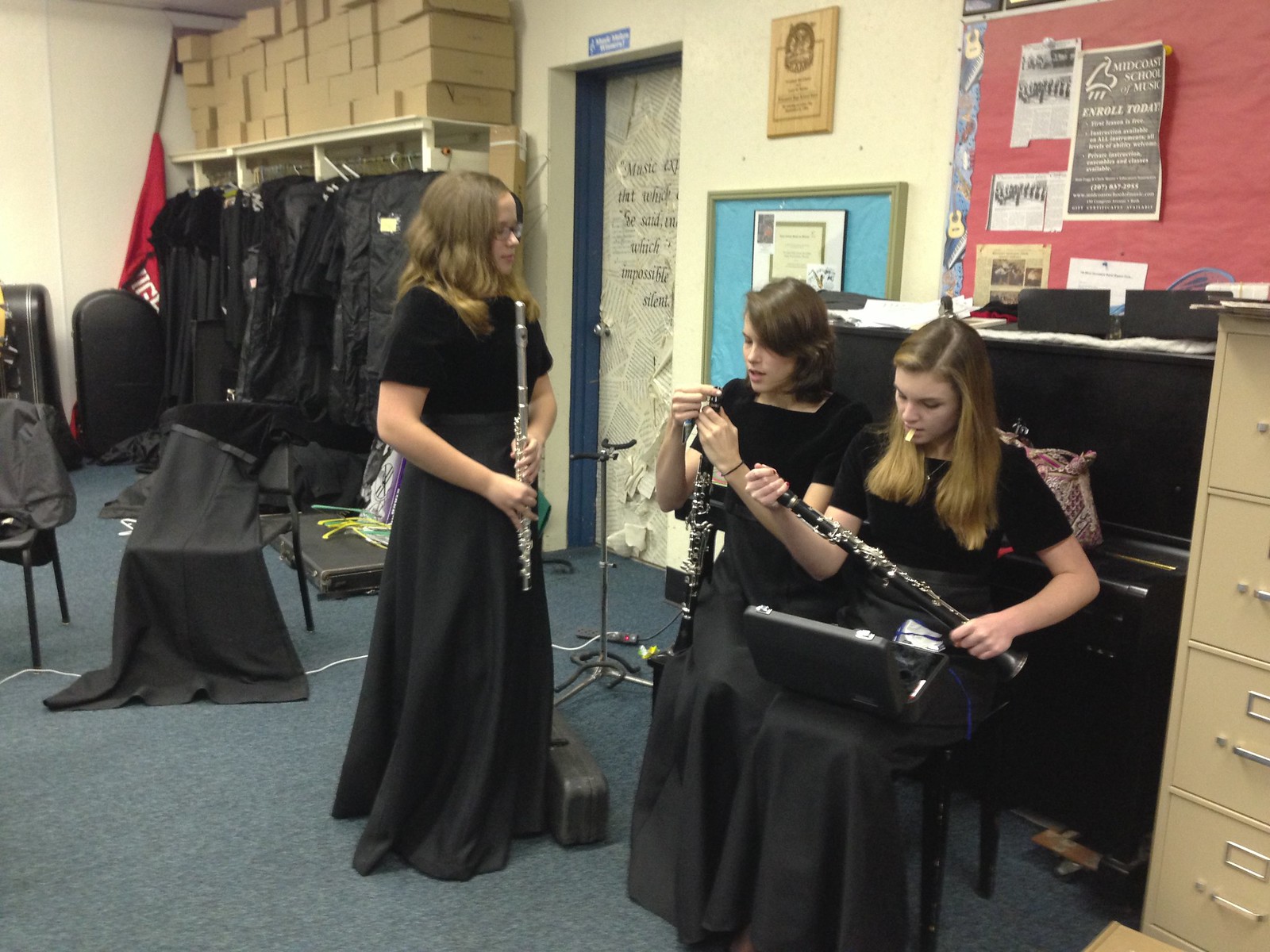In a spacious music classroom adorned with cabinets, bulletin boards, and covered uniforms, three young white girls, all dressed in long flowing black dresses, are engaged with their musical instruments. The two seated girls, each holding black clarinets, are preparing their instruments: one is in the process of cleaning or adjusting her clarinet's reed, while the other already has her fully assembled clarinet in hand, with its case resting on her lap. To their side stands a blonde girl with glasses, holding a silver flute close to her mouth. The photograph, captured in a landscape orientation, beautifully showcases the diligent preparation and focus of these young musicians prior to their practice or performance.